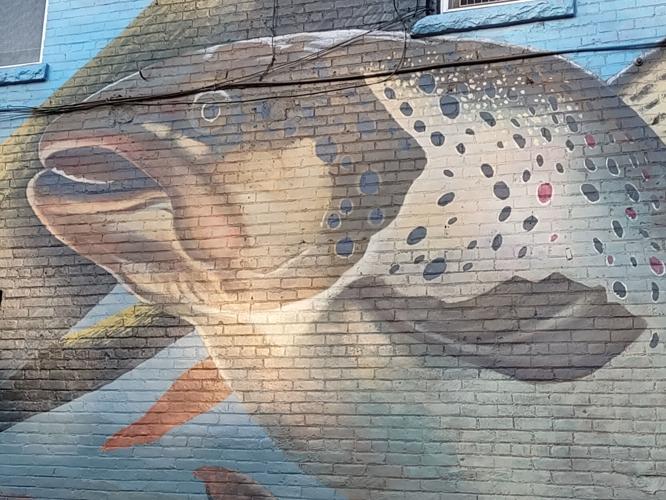The image is a wide rectangular photograph showcasing a large, highly detailed mural painted on the side of a brick building. The mural depicts a massive fish, primarily brown in color, with its head positioned toward the upper left corner of the wall. The fish's open mouth and single visible hazel eye give it a vivid expression, while its body transitions from brown to a cream or white color toward the center and right edges. The fish's detailed pattern includes numerous dark blue, red, and black spots, especially noticeable near its head and body. A prominent brown fin is visible near the center. The brick wall hosting the mural alternates between thin rows of tiny rectangular bricks. In the upper portions of the wall, there are partially visible windows; the top left shows the bottom right corner of a window with a grey screen and a blue brick underneath, whereas the top center features another window with a grey grate and another blue brick below. The background of the mural includes light blue patches and what appears to be a depiction of branches or a tree featuring shades of brown and hints of green. Additionally, a crack runs along the brick wall just below one of the windows, adding to the wall's textured appearance.